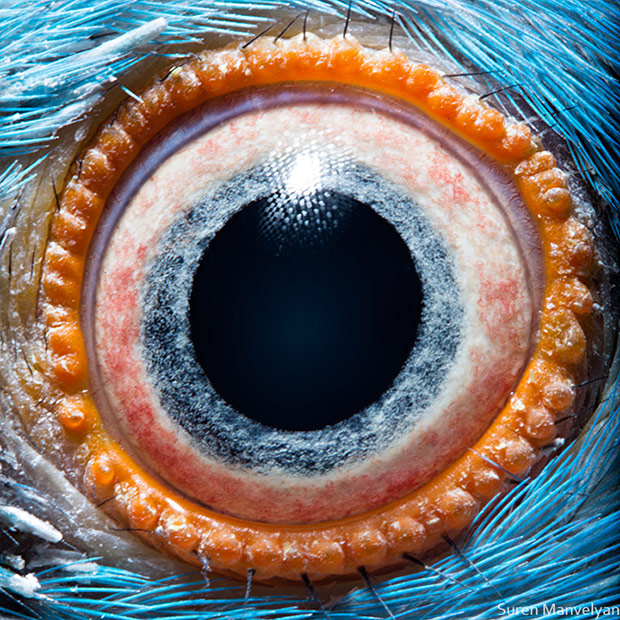The image displays an extremely close-up view of a bird's eye, presented vertically without specific borders or a discernible background. Dominating the center is a large, perfectly round, black pupil that catches a glint of light at the top. This pupil is encircled by a narrow band of light gray, which seamlessly transitions into the sclera, a predominantly white area infused with red streaks. Surrounding the sclera is a prominent bumpy orange ring adorned with fine, black hair-like protrusions. The outermost layer features short, overlapping blue feathers that create a delicate, textured pattern, emphasizing the avian origin of the eye. The combination of hues—black, gray, red, orange, and blue—along with the intricate details of feathers and hair, forms a striking and detailed portrait of the bird's eye.